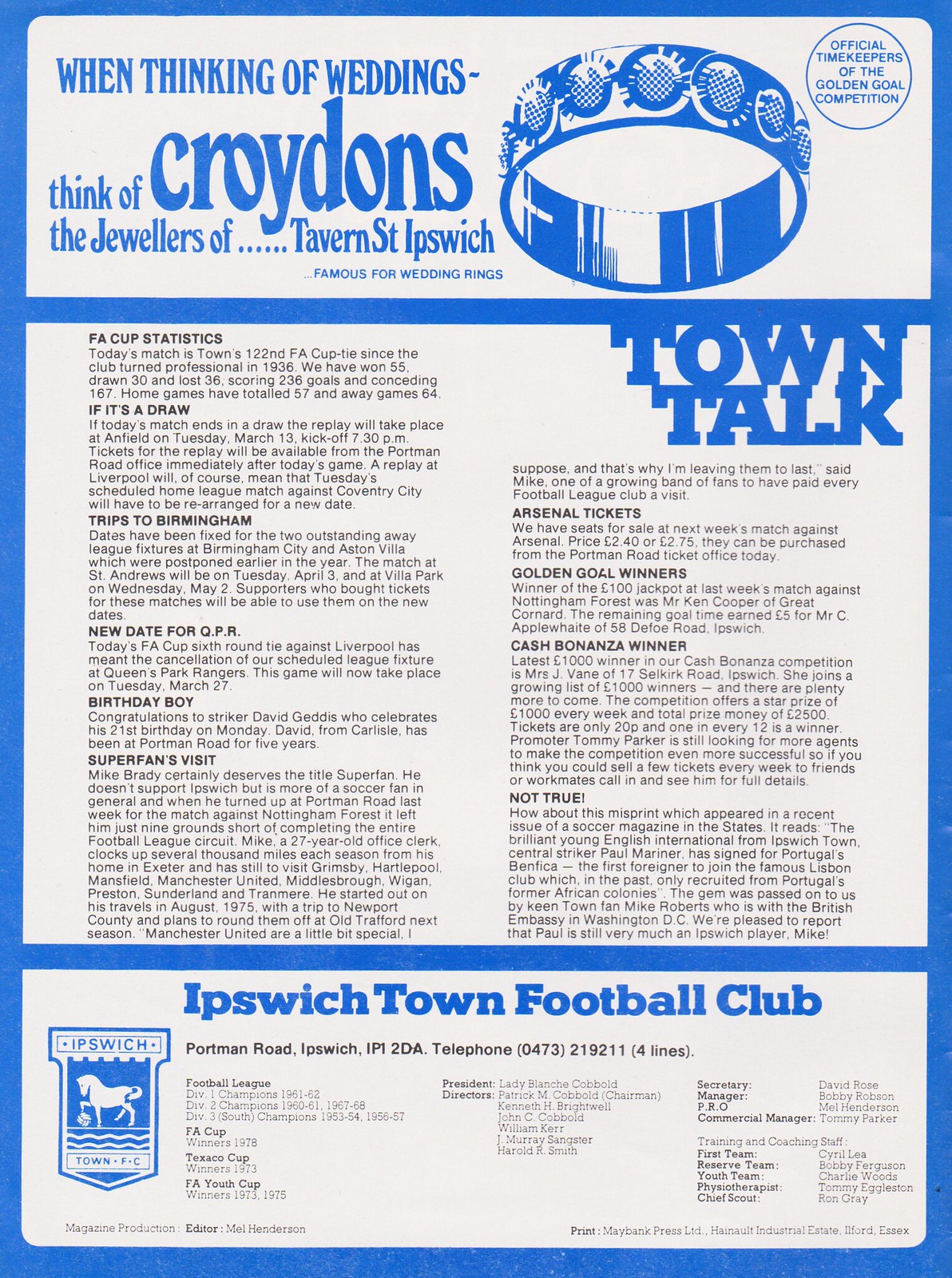This poster, with a light blue background and a blue border, serves as an advertisement and an informational page. Dominating the top section, in blue text, it reads, "When thinking of weddings, think of Croydon's, the jewelers of Tavern St. Ipswich, famous for wedding rings." Next to this tagline, a striking image of a jeweled wedding ring is prominently featured. To the upper right of this image, enclosed within a circle, the text announces Croydon's as the "Official Timekeepers of the Golden Goal Competition."

Below this section, a blue bar spans the width of the poster, dividing the advertisement from the main content area. Here, in large blue letters, it states "Town Talk," followed by numerous paragraphs of detailed information about various topics. The larger part of the content includes FA Cup statistics, updates on match results, potential replays, rescheduled fixtures against teams like Coventry City, Birmingham City, and Queen’s Park Rangers, and an acknowledgment of striker David Giedis’s 21st birthday.

Additionally, there are noteworthy mentions such as a superfan named Mike Brady's extensive travels to various football grounds, Arsenal ticket sales, last week's Golden Goal competition winners, and the latest Cash Bonanza prize winners. The section also humorously corrects a false report about a player transferring to Benfica.

At the bottom, another blue bar demarcates the promotional content from the official club information. Here, it states in blue letters, "Ipswich Town Football Club," and lists significant contact details, achievements, and key personnel within the club, from the President to the training and coaching staff, cementing its comprehensive nature.